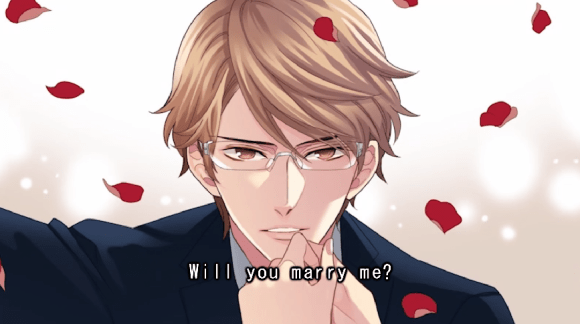The image is a detailed cartoon depicting a male character, with light brown, wavy, and layered hair, wearing thin-rimmed glasses and a dark blue coat. He has a fair, pinkish-white complexion and light brown eyes. The man is facing the viewer, with his hands raised towards his chin where they are clasping another person's hand. The scene is set against a predominantly white background with subtle pink and light gray hues, and red rose petals are falling around the character. The lighting source is from the right, casting a shadow on the left side of his face. At the bottom middle of the image, the text "Will you marry me?" is written in white letters with a black outline.